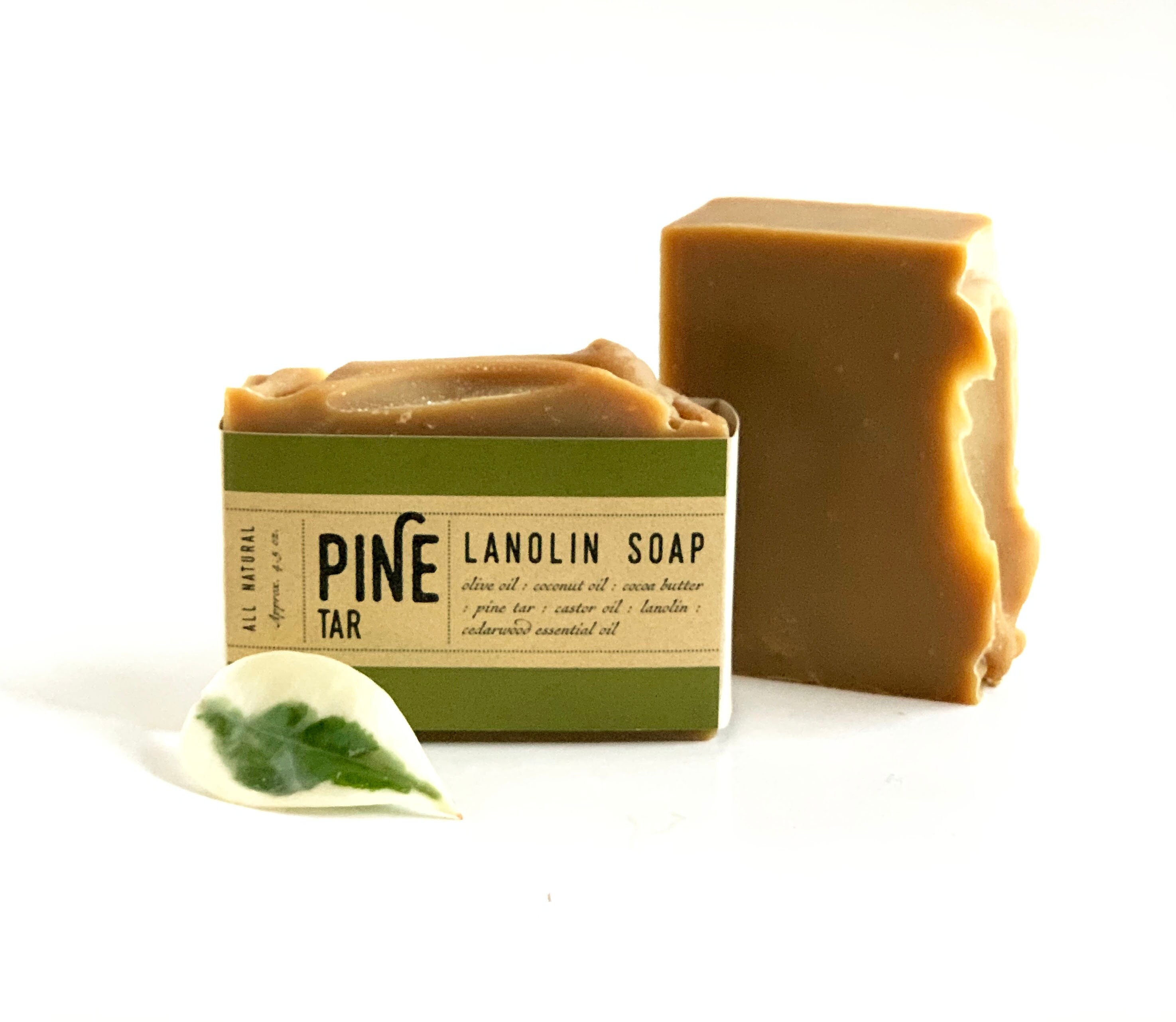This color photograph features a distinctive bar of lanolin soap against a stark white backdrop. Central to the composition is a caramel brown bar of soap lying on its side and adorned with a green and brown cardboard label. The label is detailed with the words: "All Natural, Pine Tar, Lanolin Soap, Olive Oil, Coconut Oil, Cocoa Butter, Pine Tar, Castor Oil, Lanolin, Cedarwood Essential Oil." Notably, there is a small leaf icon on the front of the label, white with vibrant green veins. To the right, another bar of the same soap stands upright on its jagged, uneven edge, as if it was broken from a larger piece. The rustic appearance of the soap, with its homemade aesthetic and rugged edges, juxtaposes with the polished packaging, highlighting its all-natural ingredient list and artisanal feel.